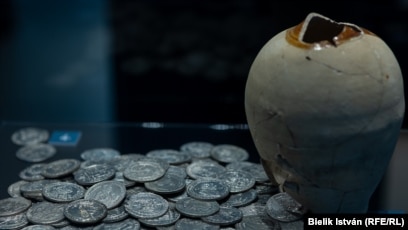The image depicts a small, oval-shaped ceramic jar, resembling an antique piggy bank or money jar, with a distinctive gray hue and a brown, circular rim around its mouth. The jar appears aged, with cracks and a broken top, suggesting it was recently broken open. Scattered beside the jar on the left side is a sizeable pile of silver, shiny coins, resembling quarters, though they may be foreign. The background is very dark, possibly a black wall or door, and in the bottom right corner of the image, white text reads "BIELIK ISTVAN R-F-E/R-L." The overall scene conveys an intriguing snapshot of what looks like a collection of coins spilling out from a treasured, yet time-worn, container.